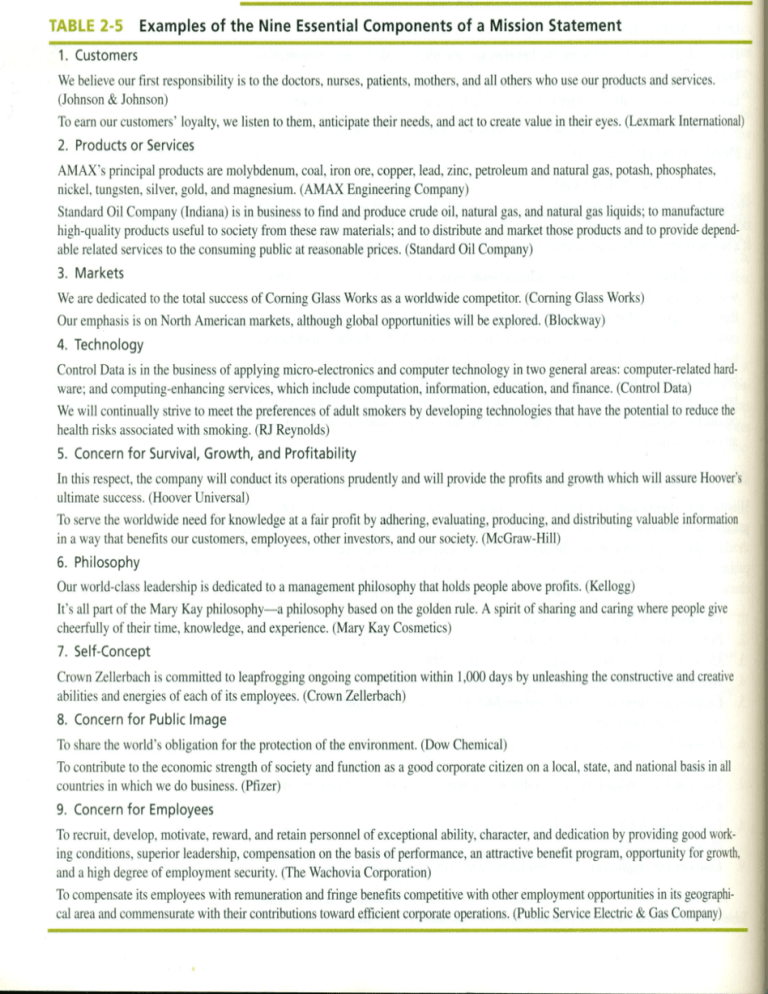The image displays a detailed table titled "Table 2-5: Examples of the Nine Essential Components of a Mission Statement." The background is plain white with black text, characteristic of a photocopy. The right side of the image appears slightly cut off while the left side is slightly curved, suggesting it might have been photocopied from a book that was pressed flat. The image includes color elements, particularly a green border beneath an untitled section, indicating it could be a color photocopy.

The table itself is organized into nine categories: 
1. **Customers** 
   - Example: "We believe our first responsibility is to the doctors, nurses, patients, mothers, and all others who use our products and services." (Johnson & Johnson)
   - Example: "To earn our customers' loyalty, we listen to them, anticipate their needs, and act to create value in their eyes." (Lexmark International)
2. **Products or Services**
3. **Markets**
4. **Technology**
5. **Concern for Survival, Growth, and Profitability**
6. **Philosophy**
7. **Self-concept**
8. **Concern for Public Image**
9. **Concern for Employees**

Each section features one or two succinct mission statements from notable companies such as Mary Kay, Crown, Zellifax, Pfizer, and Public Service Electric and Gas, highlighting distinct aspects of their corporate missions. The bottom of the image has a slight shadow, enhancing the photocopied appearance. This table serves as a resource showcasing various approaches to crafting mission statements across different business components.